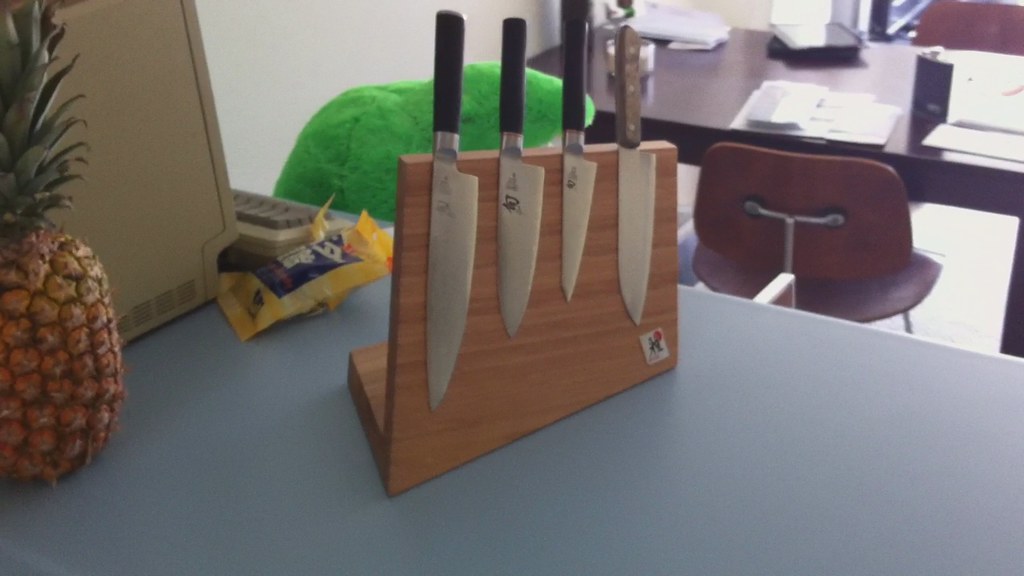This is an indoor photo of a room, possibly a school or office, featuring a meticulously detailed scene. The photo foreground showcases a blue counter with several intriguing items. Prominently, there's a magnetic knife block in an L-shape, displaying four knives—all with blades seemingly suspended. Three knives sport black handles, while the knife on the far right has a well-worn wooden handle. 

Next to this knife display rests a ripe, yellow pineapple, ready to be cut. Beside the pineapple lies a yellow open snack bag and a bright green fluffy stuffed animal, adding a playful touch. Adjacent to these items is an old-style computer monitor paired with a keyboard. In the background, the room’s white walls and floor provide a clean backdrop. A brown table can be seen at a distance, adorned with scattered papers and flanked by burgundy chairs, adding an element of organized workspace.